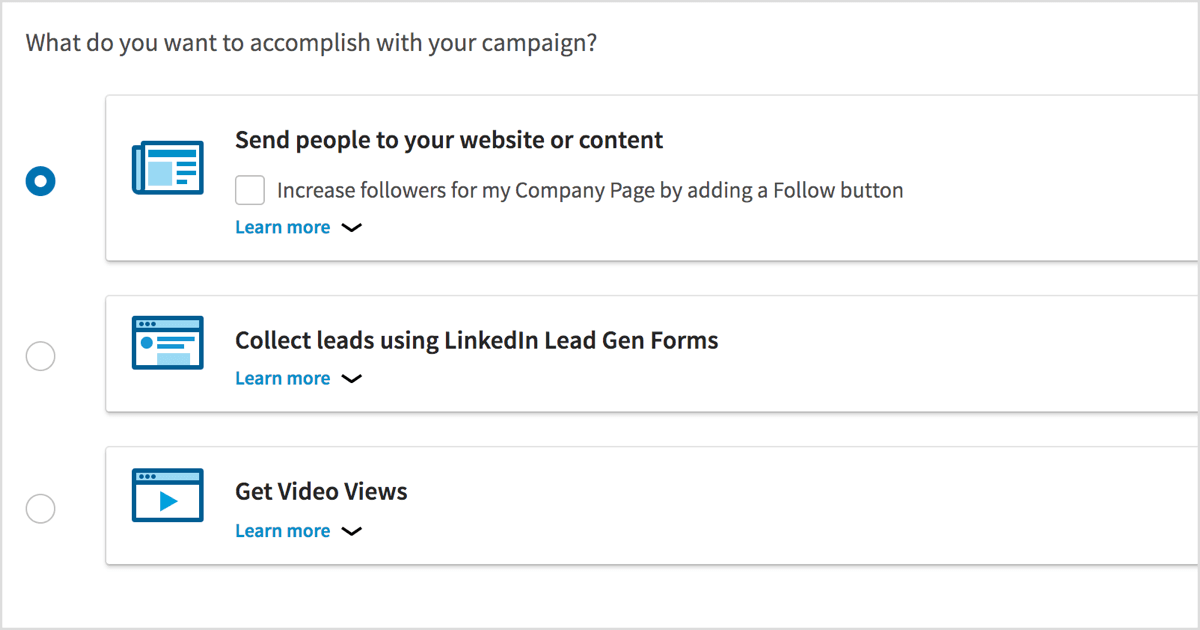This is a screenshot of a webpage or app interface, presented as a horizontally oriented, light gray rectangle located at the top left corner of the screen. The main header, set in dark gray, reads "What do you want to accomplish with your campaign?" 

Below the header, there are three outlined sections in gray, each corresponding to different campaign choices. On the left side of these sections, there are radial buttons to select an option. There are three circles in total: the top one is filled in with a blue circle containing a white center, indicating it is selected, while the other two are empty gray circles.

Starting from the top section:

1. **First Section:**
   - **Icon:** A dark and light blue icon resembling a stacked newspaper, located on the left.
   - **Text:** "Send people to your website or content," in bold black font.
   - **Additional Option:** Below, there's an unchecked square checkbox followed by the text "Increase followers from my company page by adding a follow button" in dark gray.
   - **Learn More:** "Learn more" in blue text, accompanied by a small downward arrow to the right, suggesting additional information or options can be revealed.

2. **Second Section:**
   - **Icon:** A web page-like icon with a small circle at the top left, all in shades of dark and light blue, located on the left.
   - **Text:** "Collect leads using LinkedIn Lead Gen Forms," in black font.
   - **Learn More:** Again, "Learn more" in blue text with a small downward arrow next to it for further details.

3. **Third Section:**
   - **Icon:** An icon resembling a web page with a video play button, all in shades of dark and light blue, located on the left.
   - **Text:** "Get video views," in black font.
   - **Learn More:** "Learn more" in blue text, accompanied by a small downward arrow.

Each of the icons in these sections is outlined in a dark blue, providing a clear visual structure to the interface options.